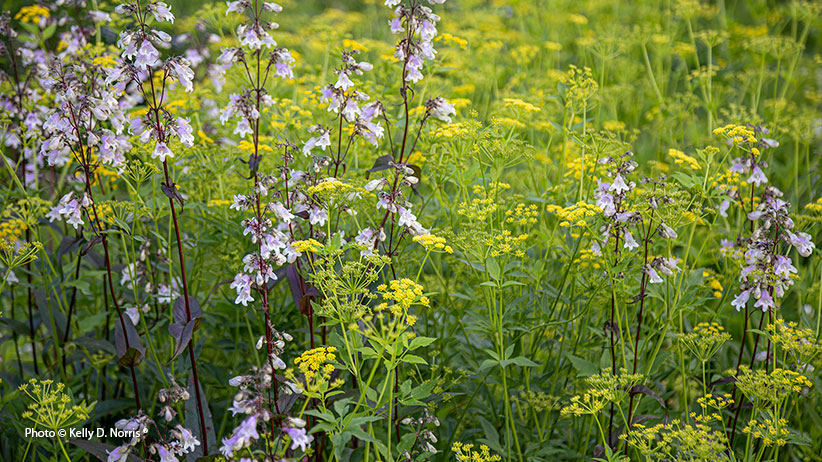This photograph captures a vibrant outdoor landscape teeming with wild plants and flowers. The foreground prominently features lush greenery, with long, tall stems adorned with green leaves. Interspersed among the foliage are clusters of striking yellow flowers. Additionally, the image showcases intriguing contrasts in color and texture, as some flowers boast tall, dark brown to blackish stems and have leaves of a dark hue. These darker stems support flowers that vary in shades from white to light lavender, sometimes appearing almost blue. 

While the predominantly green and yellow foliage fills most of the frame, the white and lavender flowers are more densely concentrated towards the left-hand side and sporadically on the right. The background suggests either a deep blue sky or a field of water, enhancing the natural beauty and open feel of the scene. The photograph, taken in daylight, perfectly captures this wild, untamed garden environment without the presence of people or other distractions. Notably, the only text in the image is a small, subtle credit to the photographer, "Kelly D. Norris," placed in the lower left-hand corner.